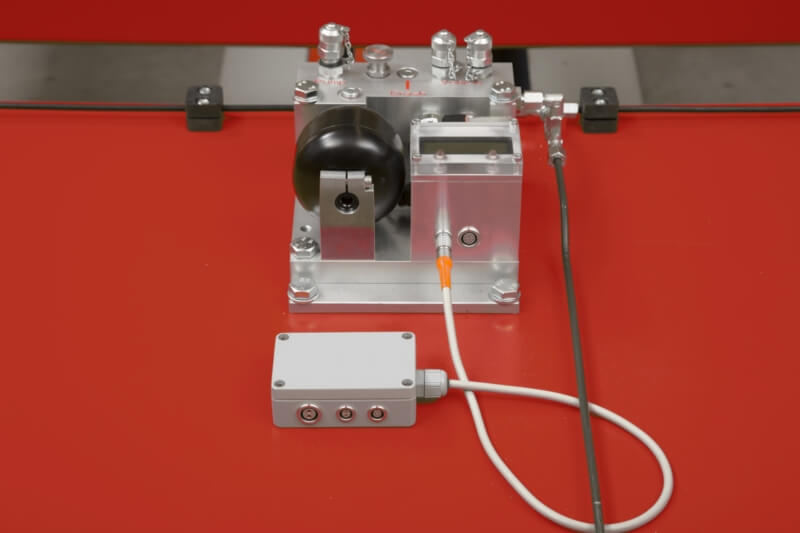The image depicts a detailed, close-up view of a small, silver piece of electronic equipment positioned on a shiny red countertop, with the reflection of the metal faintly visible on the surface. The equipment appears bolted to the countertop and features several components and connections. On the left side of the device, there is a black circular plastic piece mounted with a screw. A black hose emerges from the right side, ending in a square black plastic handle. Central to the front panel is a small white cord that extends and connects to a gray rectangular control box lying directly in front of the device. This control box includes three plug-in receptacles visible on its faceplate. The equipment itself is adorned with several silver screws and knobs, with an LED screen posited to face upward. Additionally, a dark gray horizontal strip with black clips is situated above the device, contributing to the meticulous arrangement and intricate design of this mechanical setup.